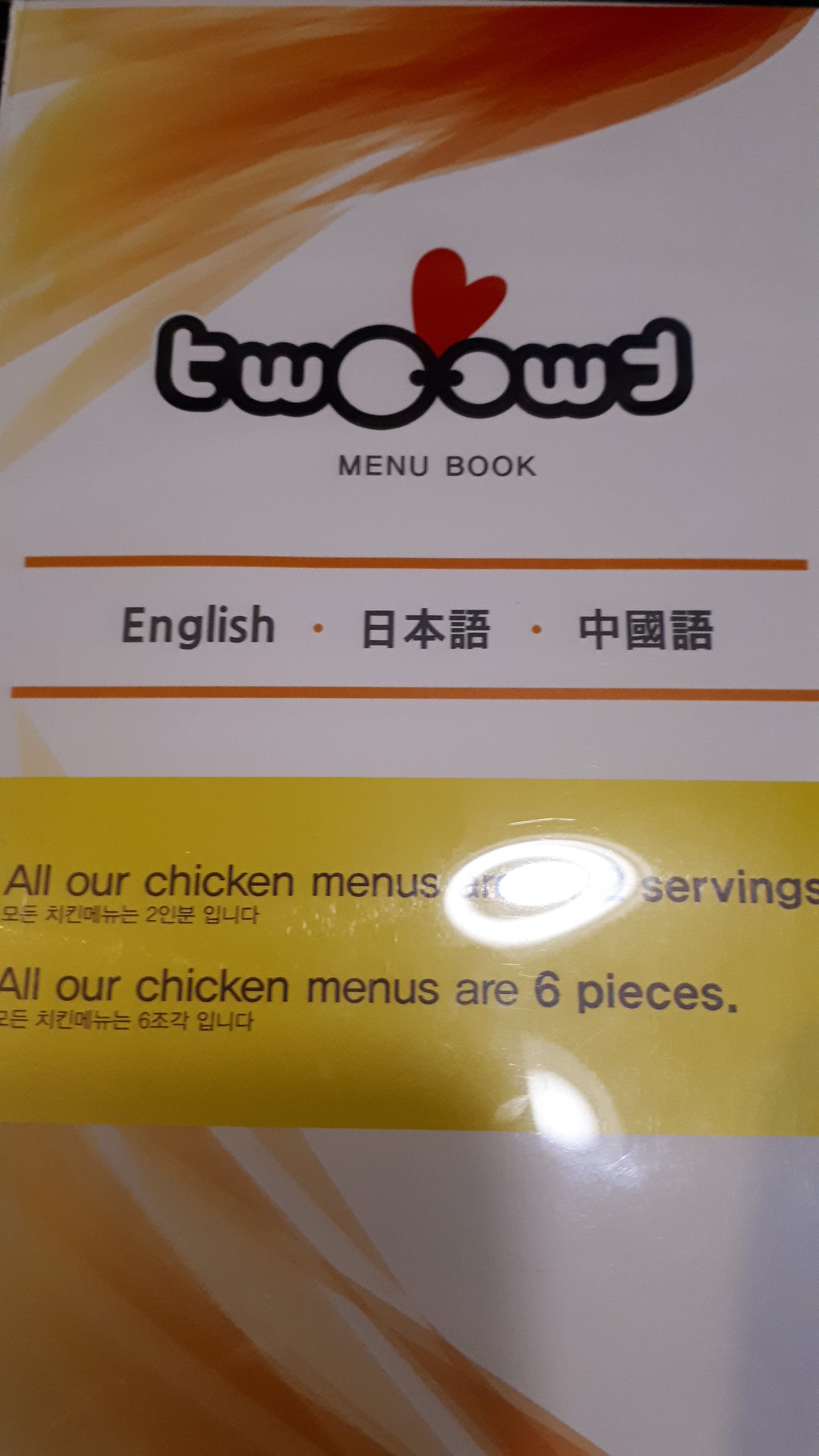The photograph appears to be taken from a cell phone and captures the cover of a glossy, laminated menu book. The cover features bubble lettering at the top that reads "TWOO*WT," with a heart shape forming from the two 'O's. Notably, the second "OWT" is a mirrored version of the first, with the 'O' slightly smaller. Below the title, "MENU BOOK" is written in plain uppercase text. An orange horizontal line separates this title from the content below.

Further down, there are three segments: "ENGLISH," an orange dot, characters that seemingly belong to an Asian language, another orange dot, and more foreign characters possibly in a different Asian script. Another orange horizontal line demarcates this section from the rest.

There is a yellow block section prominently displaying "ALL OF OUR CHICKEN MENUS." Below this heading, additional text mentions "ALL OUR CHICKEN MENUS ARE SIX PIECES," although some glare from the glossy surface renders part of the text unreadable. Multiple languages are used to describe these items, as indicated by the text in various scripts beneath the English descriptions. The surrounding area of the cover features a predominantly white background with some wispy orange coloration, adding a stylish touch to the overall design.